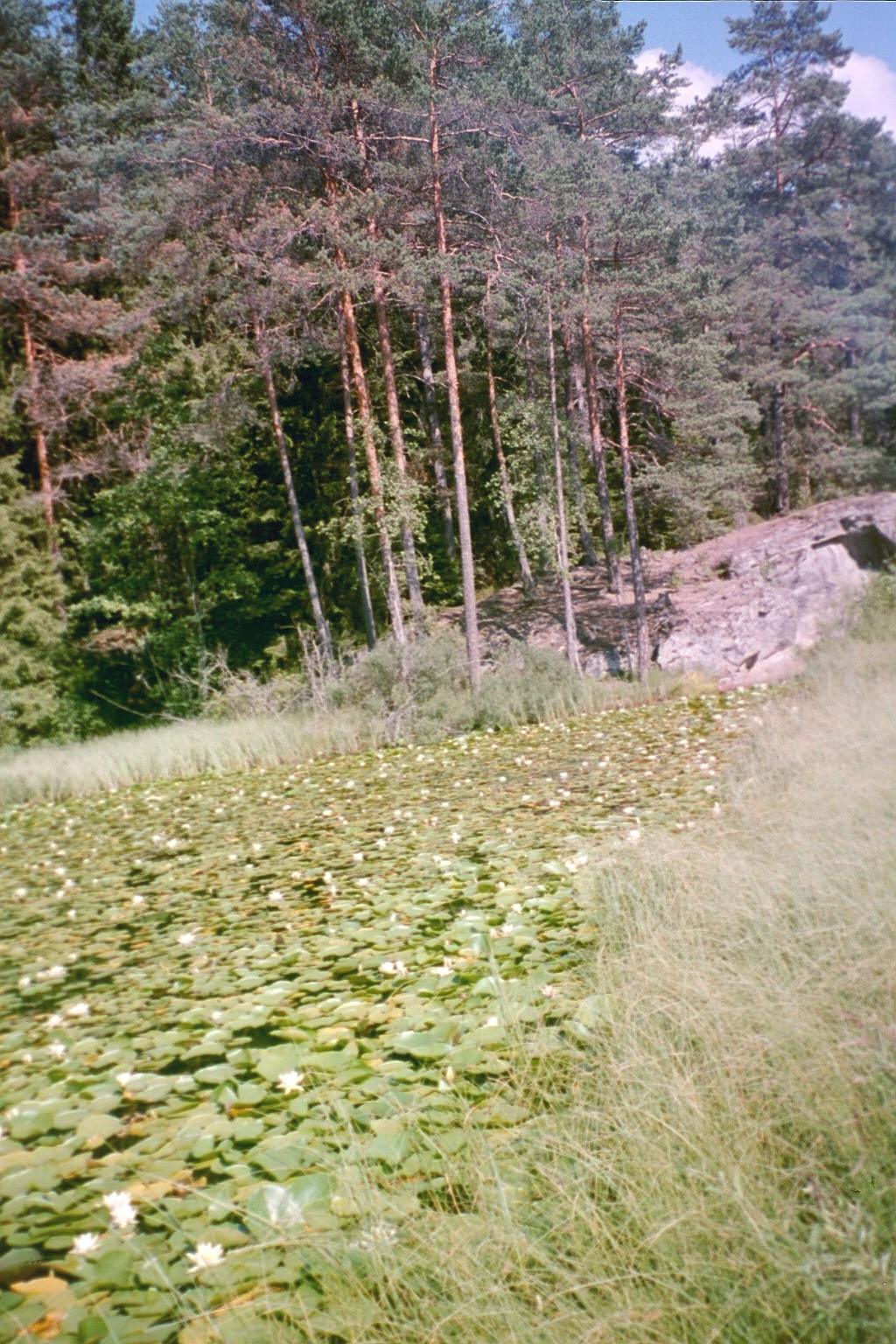The image showcases a densely wooded area with a unique foreground. In the bottom left, there is a pond completely covered with green lily pads and dotted with small white flowers, creating a lush, textured surface. This lily pond is bordered by tall grasses on the right and extends to a small rocky formation on the opposite shore. The trees in the background appear to be part of a densely populated pine forest, with the ones in the foreground displaying brownish hues, while deeper into the woods, the greenery becomes richer and more pronounced. Above, the sky is blue and flecked with white clouds which peek through the tree branches in the upper part of the image. The pond's edge transitions into some greener grassy patches next to a small dirt hill. Toward the background, a human figure, possibly taking a picture with outstretched arms, adds a scale of solitude and contemplation to the serene, forested landscape.